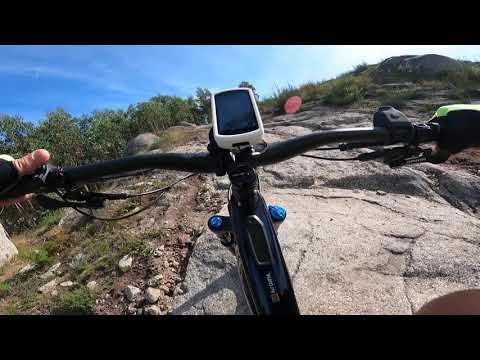The image captures the rider's perspective over the handlebars of a mountain bike, likely an electrically assisted bike given the presence of a white-bordered display panel in the middle of the black handlebars and an array of controls. The rider's left hand, adorned with a fingerless glove, rests on the left grip while the right hand, in a black glove with green accents, operates switches on the right grip. Black cables run from the center to the outside of the handlebars.

The bike navigates rugged, gray rock terrain on the side of a mountain. The left side of the scene features steep dirt with sparse green vegetation and loose rocks, while the upper right corner reveals the tallest, solid rock part of the mountain. In the background, the left side transitions into thick vegetation and a tree line, with the sky appearing mostly white except for a bright blur from the sun on the right. It is mid to late afternoon as suggested by the shadows. The camera, likely mounted on the rider's chest, captures him ascending toward the sun on a challenging, rocky path.